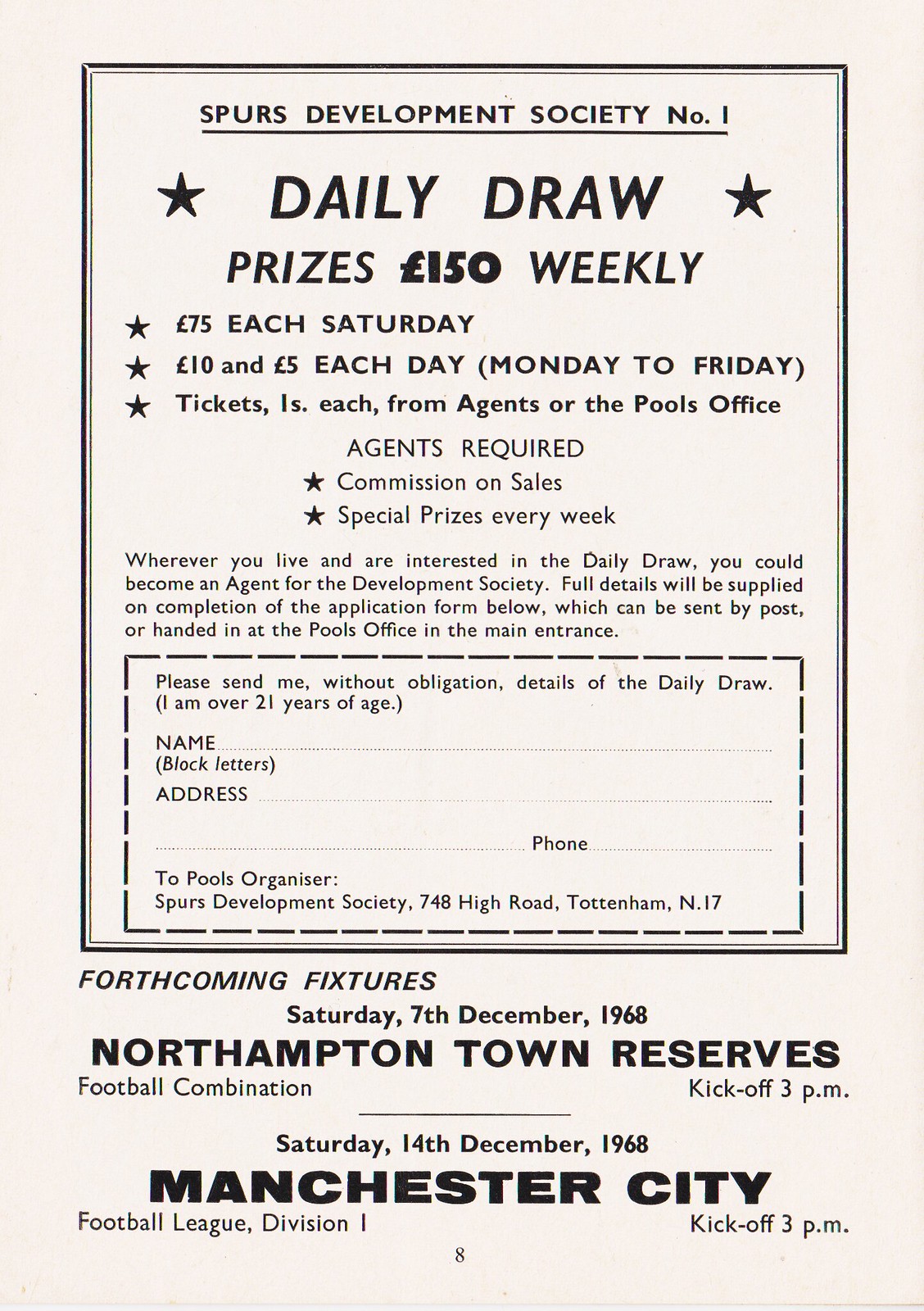The black and white poster prominently features a black outlined box at the top, highlighting "Spurs Development Society No. 1." Below, the details of the "Daily Draw" are displayed, emphasizing the weekly prize of £150, with additional prizes of £75 each Saturday, and £10 and £5 each day, Monday to Friday. Tickets cost one shilling each, available from agents or the pool’s office. There is a call for agents, stating the commission on sales and special weekly prizes. Further down, an application form invites those over 21 interested in participating or becoming agents to fill in their name, address, and phone number. It specifies the form can be mailed or handed in at the pool’s office. The bottom portion of the poster details forthcoming fixtures with bold, large text for specific events: Saturday, 7th December 1968, featuring Northampton Town Reserves in the Football Combination, and Saturday, 14th December 1968, featuring Manchester City in the Football League Division I, both with a kickoff time of 3 p.m. The entire content, including a notable black "8" at the bottom, is presented on a white background.